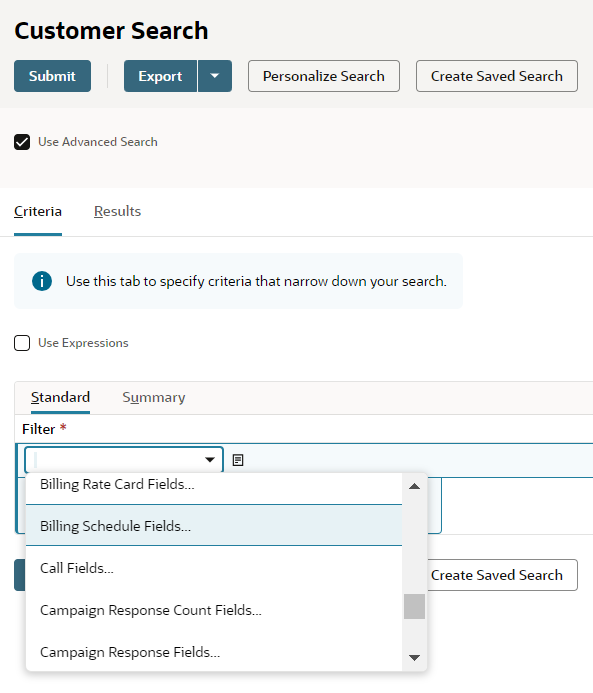The image features an all-white background with various UI elements arranged in a structured format. 

In the top left corner, bold black text reads "Customer Search." Directly below this header, there is a blue tab with white text saying "Submit." Adjacent to it, towards the right, there is a gray tab with black text labeled "Reset," separated by a vertical dividing line. Further right, another gray tab with black text says "Export," which includes a drop-down icon. Continuing along this row, the next black text on a gray background states "Personalized Search," followed by a final tab labeled "Created Saved Search."

Underneath the "Submit" button, a white box includes a blue checkmark next to the text "Use Advanced Search." A thin dark blue border separates this section. On the left side of the blue border, the text reads "Criteria," while on the right it says "Results." Below this, in smaller black lettering, it reads "Use this tab to specify criteria that narrow down your search."

Within this section, to the left, there's a white square labeled "Use Expressions." A gray border runs down the left side with the bolded text "Standard," and to the right of it, the word "Summary." Below this, red asterisks precede the words "Filter" and "Description."

Further down, there is a white-bordered box with the text "Is Customer" on the right and "Stage" on the left. This is followed by a long white tab featuring a search bar with multiple drop-down fields (seven in total) that can be clicked, each in black lettering. To the left of this search bar, a bit of a blue tab is visible with the letters "ST," and to the right, a snippet of a gray tab showing the letter "E." Another gray tab to the far right, with black text, reads "Create Saved Search."